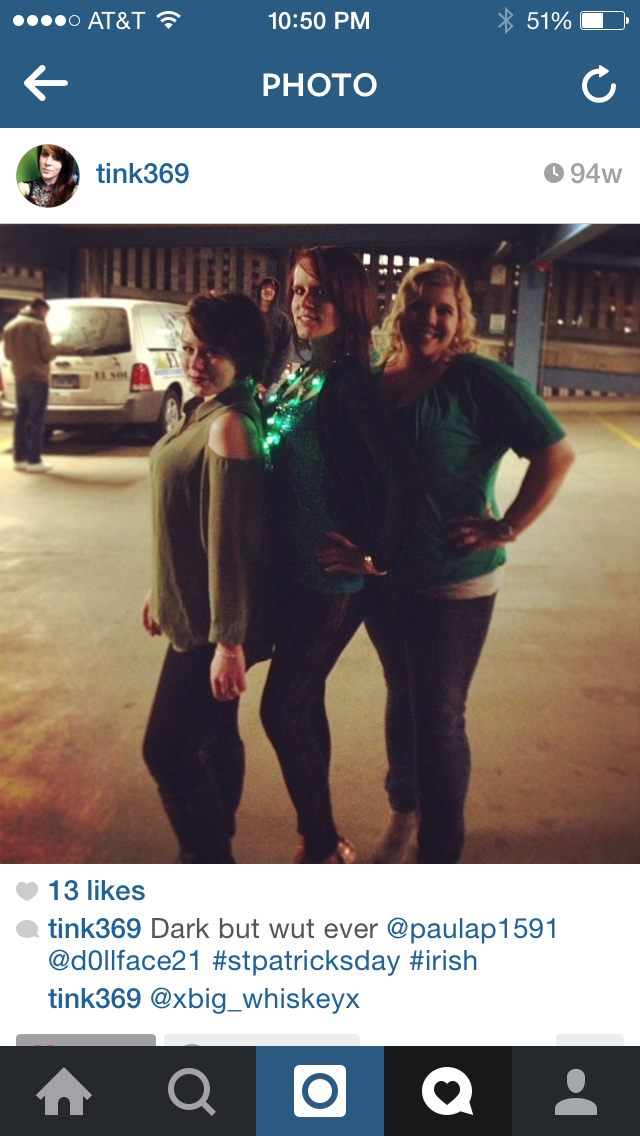This is a detailed screenshot from a cell phone displaying an Instagram post. At the top, the status bar showcases the AT&T network, a Wi-Fi symbol, the time (10:50 p.m.), a Bluetooth symbol, and a battery level of 51%. Directly below this, the app interface features the header with "PHOTO" in white text. The user's profile info follows, including a profile picture of a woman and the username "tink369" accompanied by a time stamp indicating the post is 94 weeks old. 

The main content is a photo depicting three women posed in a parking lot. All three women are dressed in green tops and jeans, with the tallest woman in the middle sporting a lit-up necklace. The woman on the left has shorter dark hair, and the woman on the right is blonde. In the background, a van and a man are visible, suggesting the photo was taken in a parking deck. 

Engagement details under the image include 13 likes represented by a blue heart icon and a comment section where tink369 remarks, "dark but whatever," tagging @paula_p1591 and @dollface21. The caption ends with hashtags "#StPatricksDay" and "#Irish," followed by the user handle 'x_big_whiskey_x', emphasizing the celebratory context of the picture.